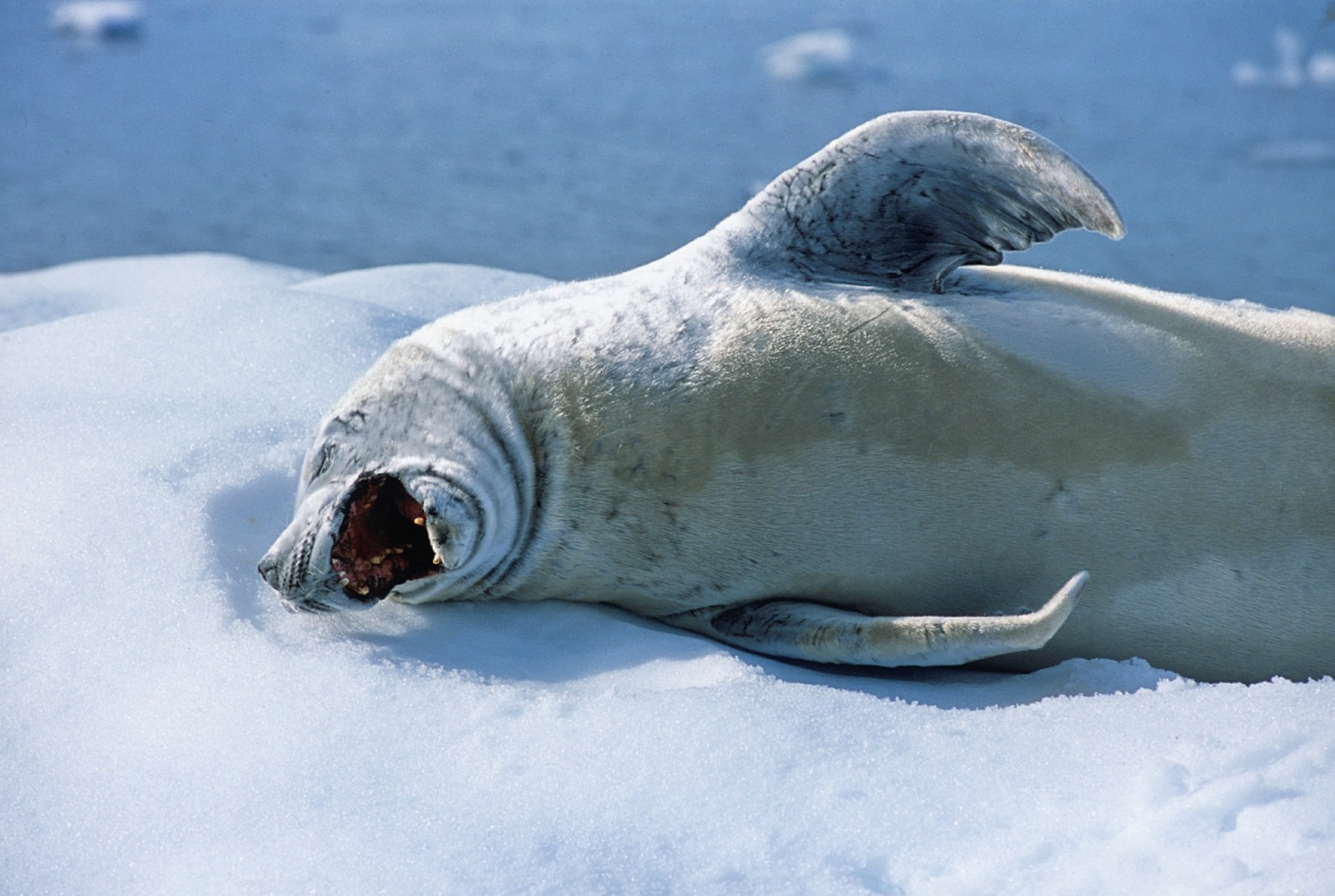In this captivating photograph, a seal is depicted lying on its right side atop a pristine, snow-covered iceberg. Its mouth is wide open, revealing sharp canines and a dark interior, creating an impression as if the seal is either yawning or emitting a loud call. The seal's eyes are closed, further enhancing the sense of a leisurely yawn. One of its flippers is raised, while the other supports its rotund body, showcasing the natural folds of fat around its neck. The seal's coat is an intriguing palette of brown and white, with a distinctive grayish-brown hue on its belly. The background features a scenic expanse of open water dotted with small chunks of ice or possibly rocks, adding depth to the chilly, yet serene environment.